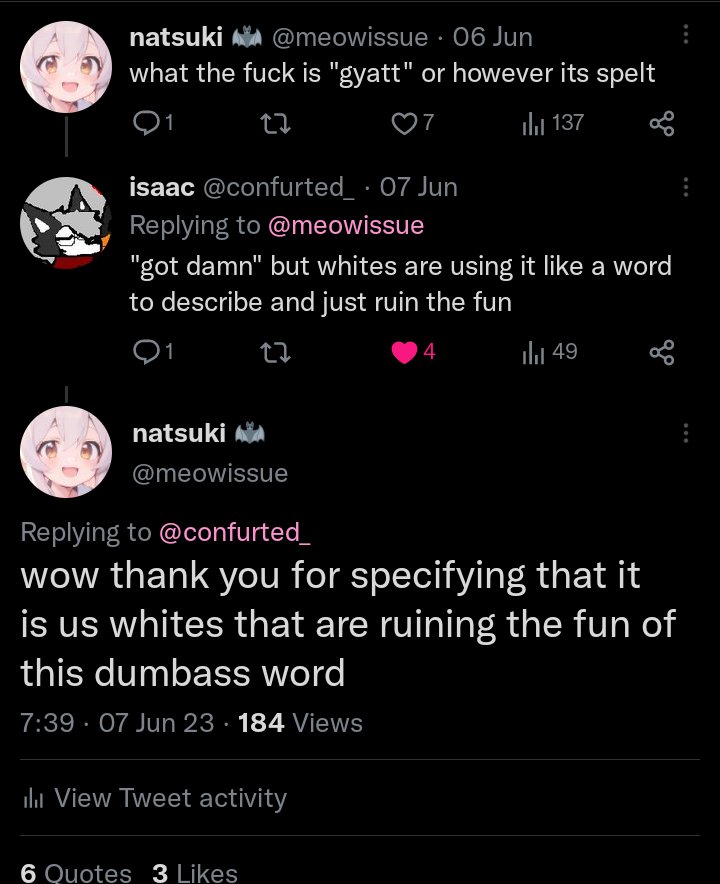In this detailed capture, we observe a social media interaction featuring a post by the user Natsuki, uploaded on June 6th. The post queries the meaning and correct spelling of the word "gyat," reflecting the user's confusion with a bluntly phrased, "What the fuck is gyat, or however it's spelled?" The post has gathered notable engagement, displaying 184 views, 6 quotes, and 3 likes.

The comment section reveals a reaction from another user who expresses frustration, stating, "god damn, but whites are using it like a word to describe and just ruin the fun." This remark appears to criticize the perceived misuse of the term by white people, suggesting it diminishes its original context or enjoyment.

Natsuki responds to this comment on June 7th, sarcastically thanking the commenter for specifying that it is "us whites" who are allegedly spoiling the enjoyment of the "dumbass word." This exchange highlights a mixture of cultural commentary and personal indignation, encapsulated within a snapshot of online discourse.